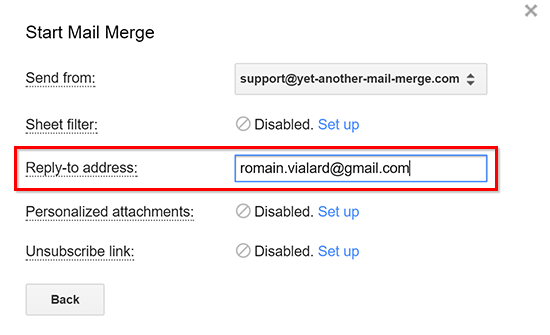Screenshot of a Mail Merge Software Interface:

In the upper-left corner, the most prominent text reads "Start Mail Merge" in the largest font. Below this, the line "Send From" appears, followed by a box containing an email address. The next line reads "Sheet Filter," which is currently marked as "Disabled" with a blue "Setup" link next to it. 

Further down is the "Reply to Address" label with a red box highlighting this section, accompanied by another email address. Below this, it says "Personalized Attachments," which is also "Disabled" with a blue "Setup" link next to it. 

The next line is "Unsubscribe Link," again marked as "Disabled," followed by a blue "Setup" link. At the very bottom of the image is a box labeled "Back."

The entire interface has a clean, white background, making the elements and text stand out clearly.